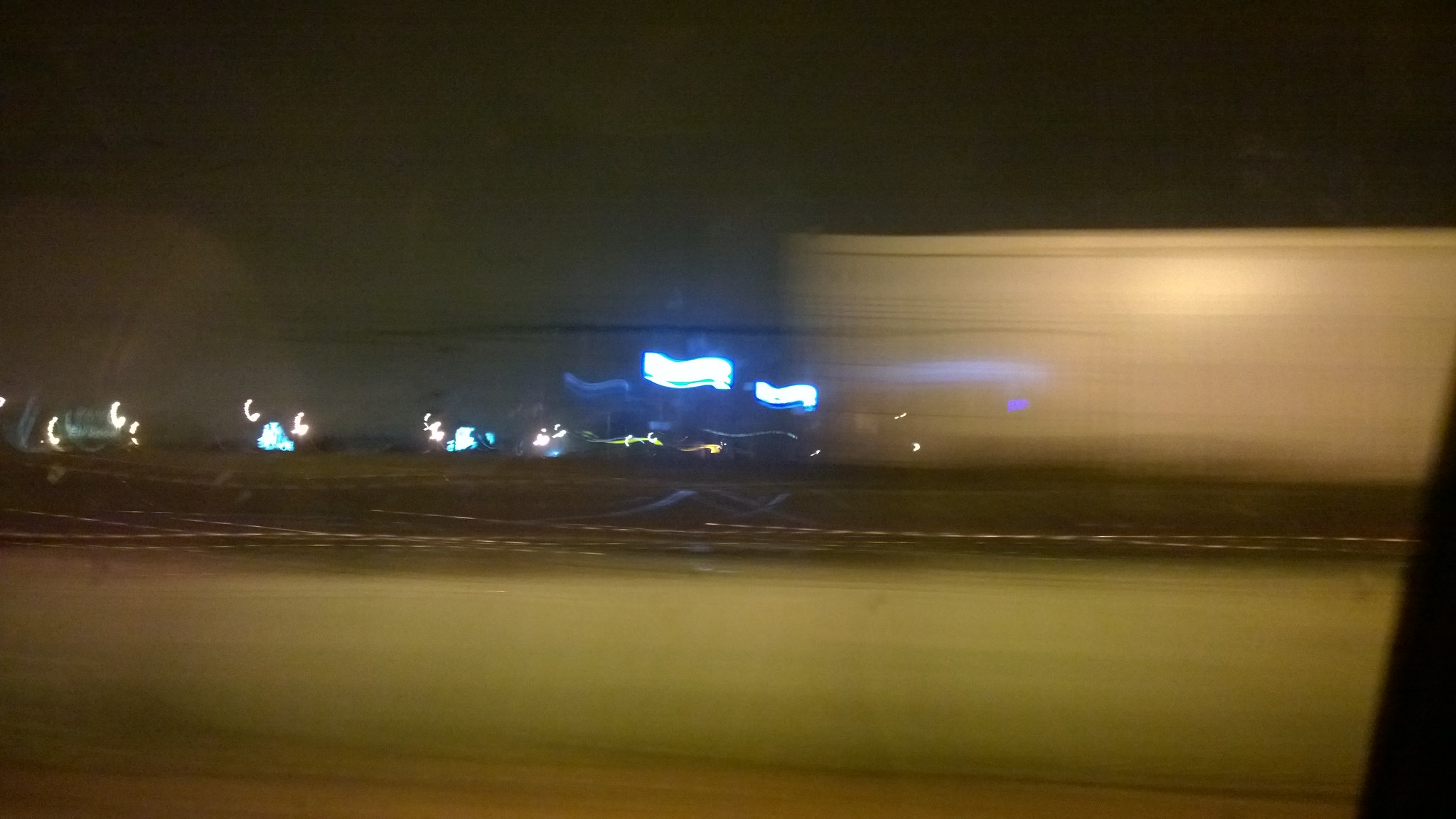This nighttime photograph, captured from within a moving vehicle, is heavily obscured by darkness and motion blur. The background is predominantly black, save for sporadic bright lights emanating from homes, buildings, or businesses visible through the vehicle's window. The glass itself reflects some indeterminate shapes, further contributing to the image's obscure quality. Notably, two streaks of blue neon lights trace across the scene, likely from a larger building or establishment, adding a jolt of color to the otherwise dark and mysterious photograph.